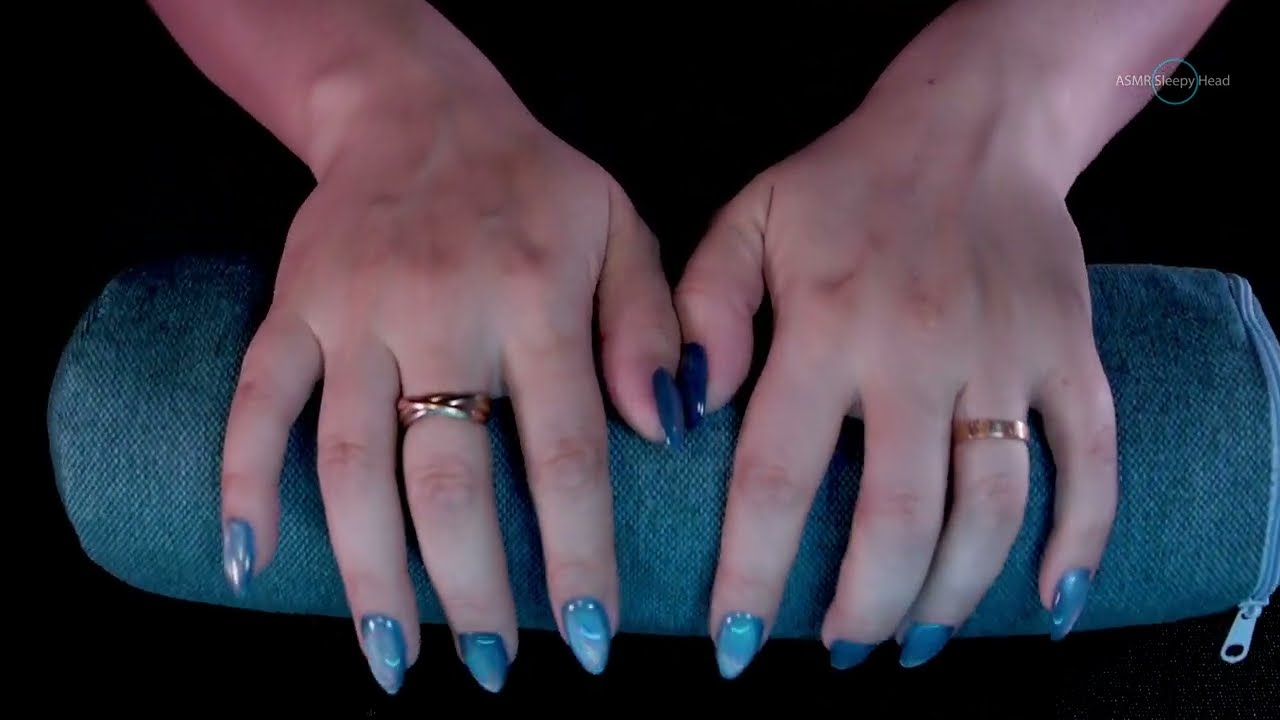The photograph captures a woman's hands resting elegantly on a light blue, cylindrical pillow adorned with a zipper and the words, "ASMR Sleepyhead" in white font, encircled by a blue ring. The hands, emerging from beyond the top of the frame, appear slightly darker than fair-skinned. Each hand is adorned with a plain gold ring, one on the left ring finger and another on the right middle finger. Her nails, professionally manicured to a pointy finish, are painted in a sky blue color with intricate white swirls that reflect the light, while the thumbs display a darker navy blue polish. The stark black background accentuates the delicate details of her hands and the blue hues of the pillow and nails.